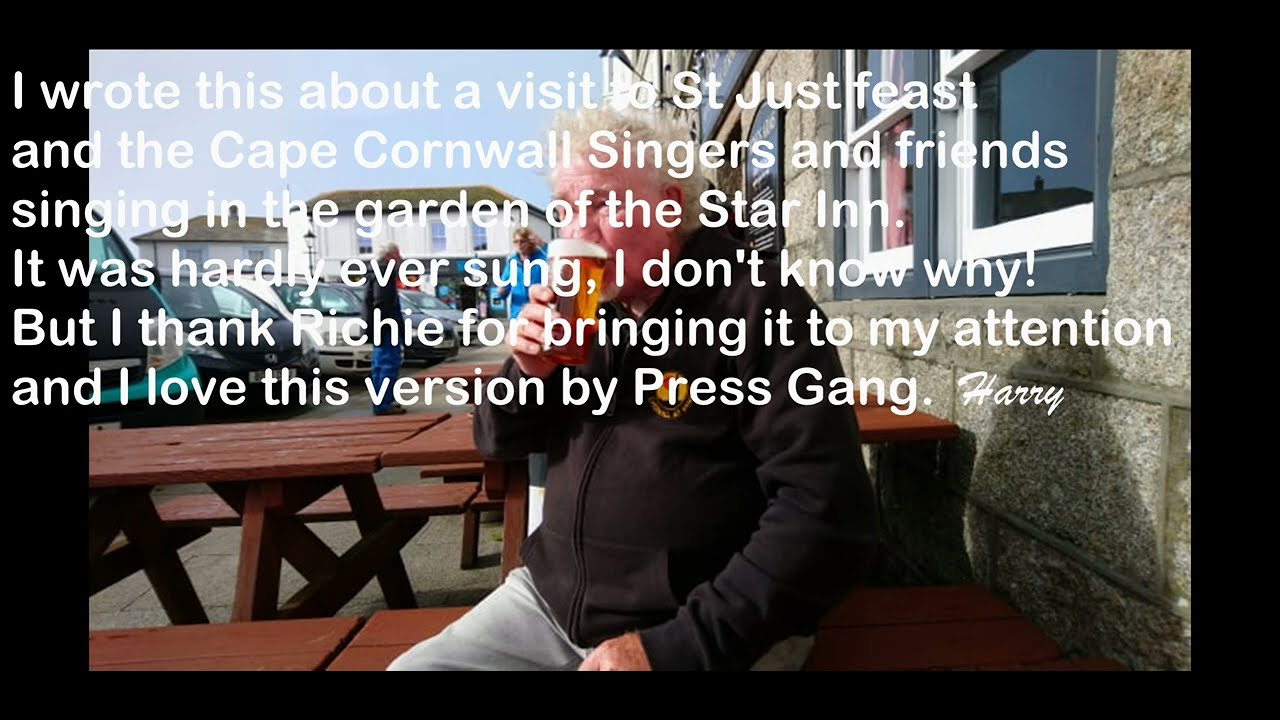A photograph captures an elderly man, possibly in his 80s, with white hair, who appears slightly overweight. He is mid-sip from a glass of amber-colored beer with a foamy top, held in his right hand. The man is seated at a brown, wooden picnic table, outdoors on a sunny day with a clear blue sky. He is dressed in a black zip-down sweatshirt and pants or shorts. The background features several picnic tables, parked cars to the left, and buildings with white sides and short, red-shingled roofs that evoke a European, potentially Germanic setting. Behind him, to the right, are windows set into a building wall. Above the image, white sans serif text reads, “I wrote this about a visit to St. Just Feast and the Cape Cornwall singers and friends singing in the garden of the Star Inn. It was hardly ever sung. I don't know why, but I thank Richie for bringing it to my attention, and I love this version by Press Gang.” Additionally, the name “Harry” appears in a cursive, brushstroke-style font next to the main text. The overall composition is framed with a black border.